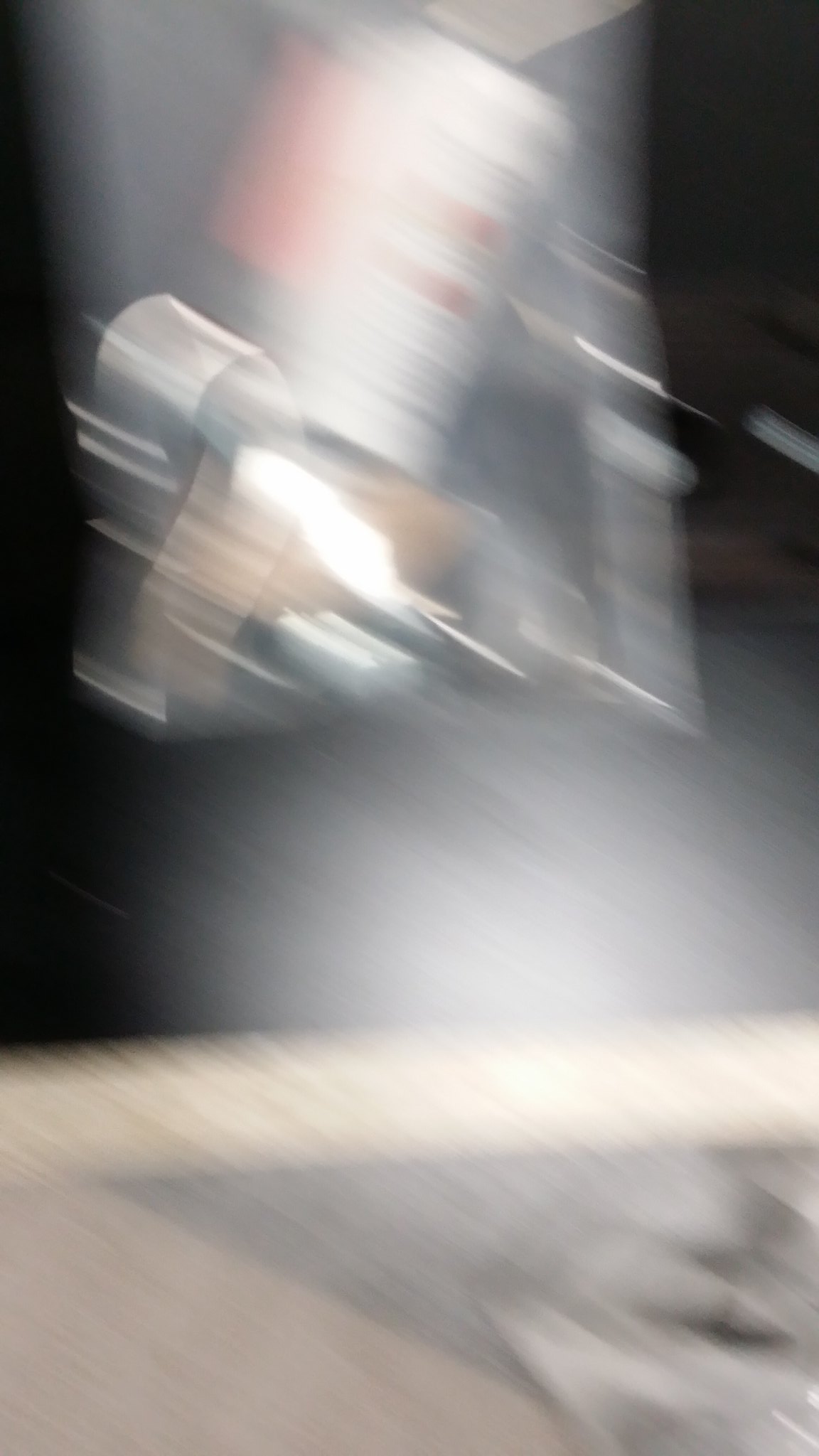The image is very blurry and highly out of focus, making it challenging to distinguish specific features. The top of the picture starts with a black area that fades into gray, leading into a bright white blur with lines running through it, possibly indicating motion. There is a noticeable diagonal white streak from left to right, creating the effect of something speeding by or a camera in rapid movement. The lower half of the image is lighter and features a larger white glare spot in the center. On the right, there's an attachment to a wall or some structure, potentially a dispenser or some dropped object like a canister with some indistinguishable writing. The bottom left shows what may be hard ground or cement. In the background, a mixture of gray and black hues can be seen with shapes that resemble tools laid on a wooden surface, which adds to the impression of a workshop setting. The entire image composition suggests a scene captured in motion, contributing to the overall disorienting blur.